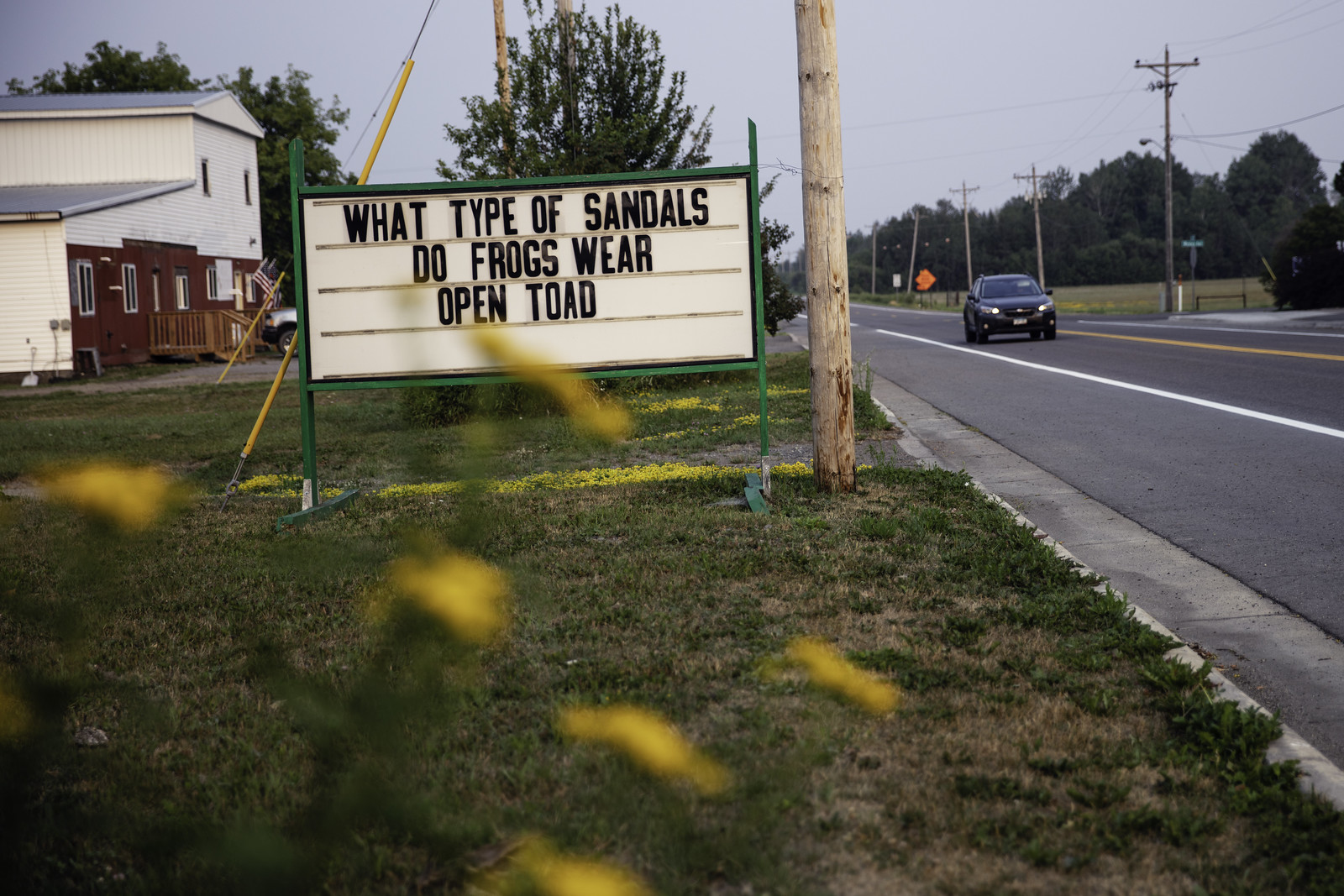This photograph captures a humorous signboard positioned on the grass verge beside a tarred road, likely taken in the early evening just after sunset. The sky is overcast with a grey hue, indicating the end of daylight, and an oncoming vehicle on the right side of the road has its headlights on, enhancing the twilight atmosphere. On the opposite side of the road, power lines stretch between poles, flanked by a field and some trees. From the photographer's vantage point on the grassy verge, yellow flowers in the foreground blur into the background, focusing attention on the comically inscribed sign.

The sign in question is mounted on a green metallic frame with a stand anchored into the grassy verge and positioned next to a wooden power pole. An evergreen tree stands behind the sign, providing a lush backdrop. To the left of the sign is a large red and white building, featuring both double and single-storey sections under a grey roof. The white sign, designed to accommodate customizable messages, asks the playful question in black block capitals: "WHAT TYPE OF SANDALS DO FROGS WEAR?" Below, the punchline answers cheekily: "OPEN TOAD." This whimsical roadside moment combines natural and man-made elements, creating a memorable and amusing scene.